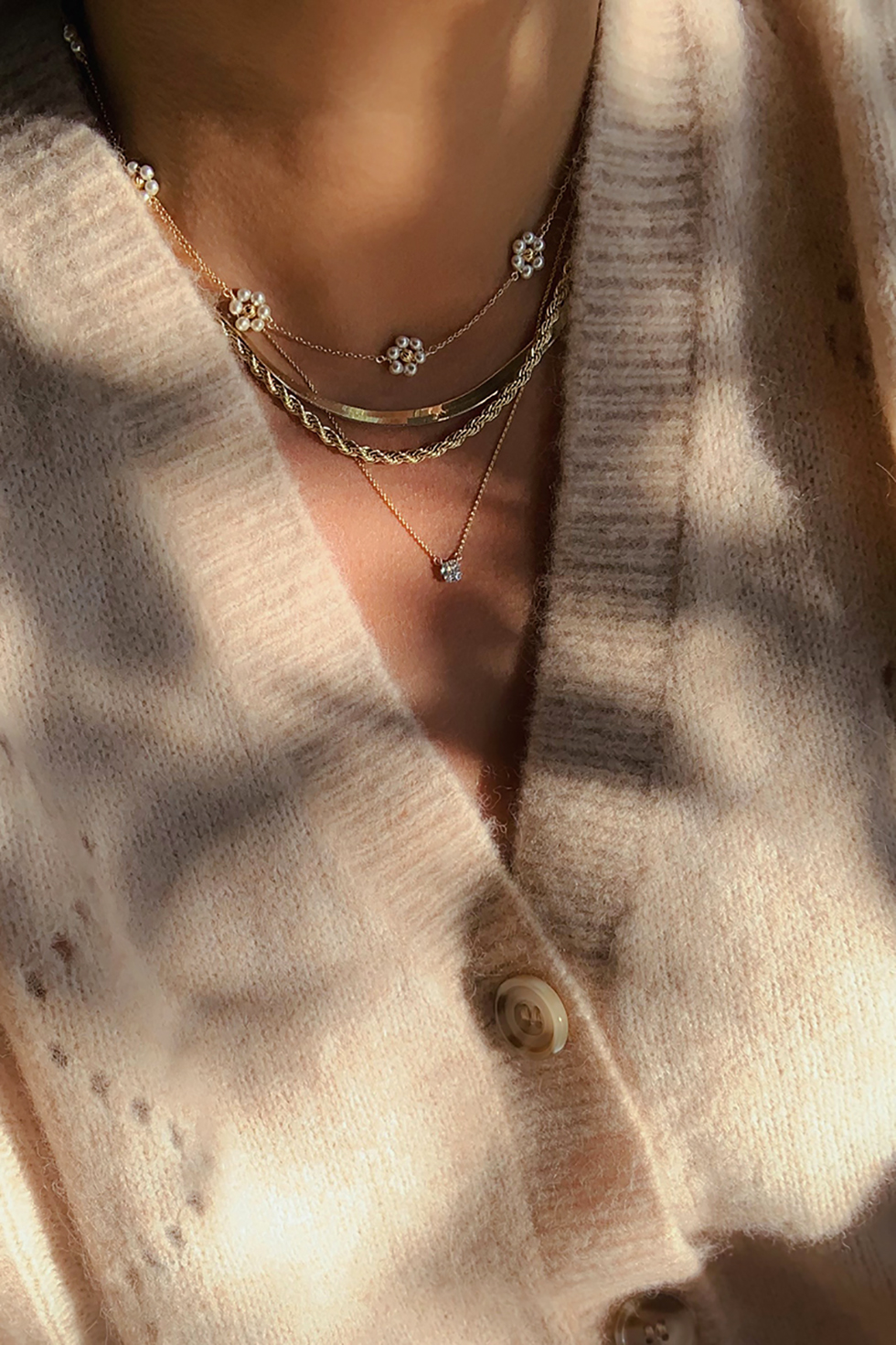This is a close-up, full-color photograph of a vertically rectangular image focused on the jewelry a woman is wearing around her neck. The picture, taken outdoors during the daytime, captures various necklaces against her light brown skin. She is wearing a button-up, cream-colored sweater with off-white, yellowish buttons, which is partially illuminated by sunlight filtering through trees, casting soft shadows on the garment.

The jewelry includes four distinct necklaces: 
1. The top necklace features clusters of seven pearls, each cluster arranged periodically with six pearls encircling a central piece, likely gold.
2. The second necklace is a delicate gold rope.
3. The third is a slightly thicker braided gold rope.
4. Finally, the bottom necklace is a thin chain with a diamond pendant.

The composition of the image, likely a professional stock photo, emphasizes the intricate details and variations of the necklaces, highlighting their arrangement against the simplicity and elegance of the woman's outfit.